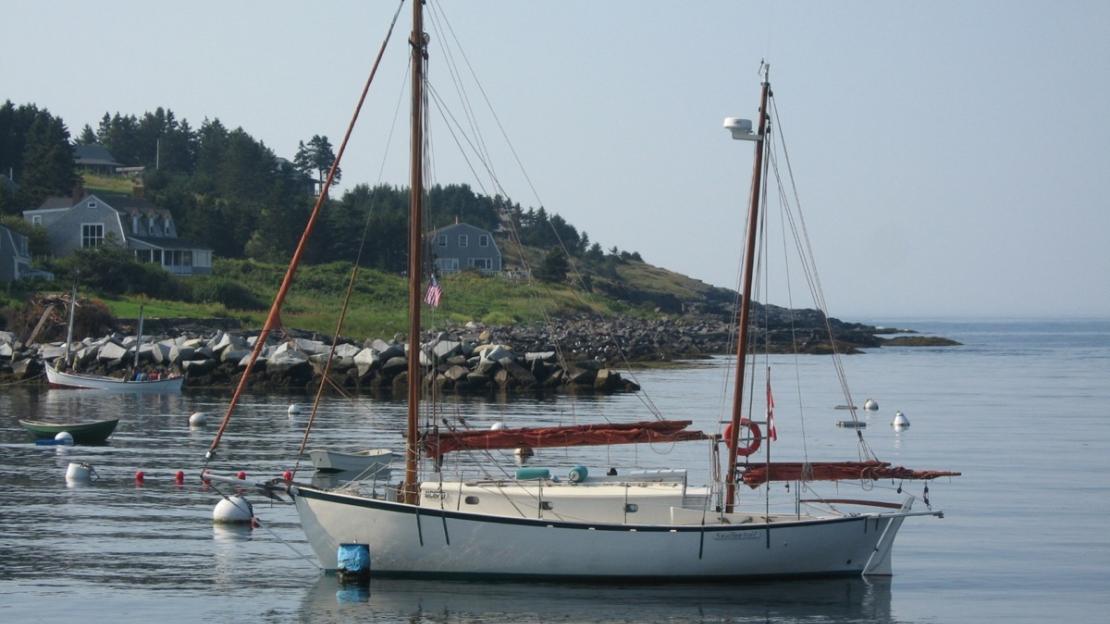A medium-sized white sailboat is docked by a barrel along a rocky shore, surrounded by buoys ideal for anchoring. This sailboat, which features three portholes below deck, has both a front and back mast with red sails currently folded down. An American flag is perched on the stern. The foreground reveals a short jetty made of rocks, with the lower portions still wet from the receding tide. The water around the sailboat is dark and murky.

In the background, we observe several houses atop a hill, associated with a coastal town atmosphere, complete with evergreen trees and green grass. These houses are a mix of Cape Cod and barn styles, displaying bluish-gray hues. A retaining wall made of large rocks lines the shore, preventing erosion. Additionally, there is another white boat in view, along with a green boat and a blue fish trap. The sky is overcast, contributing to the overall serene and slightly somber mood of the scene.